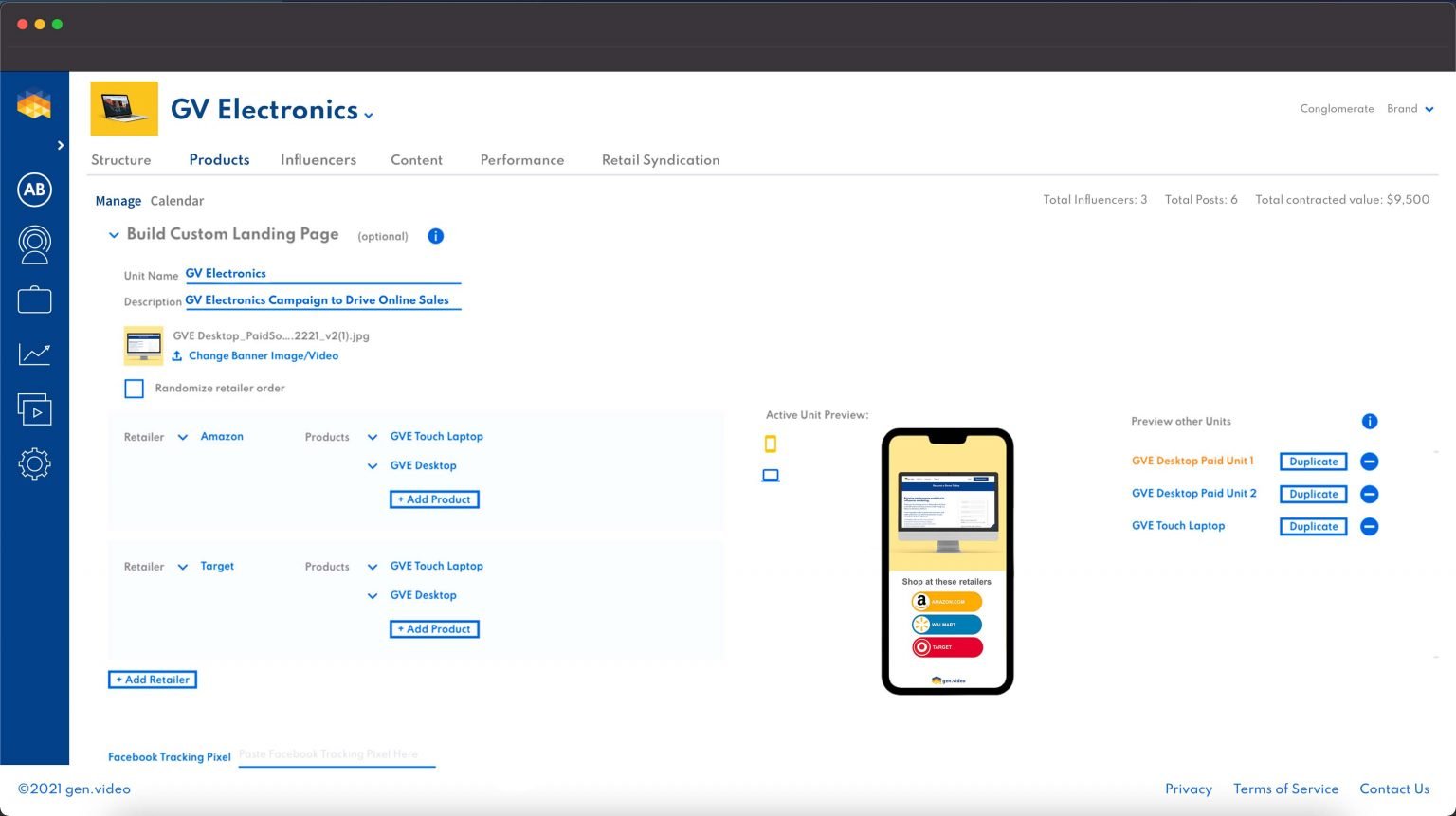Detailed Caption:

The image shows a comprehensive website design interface for GV Electronics, prominently featuring their logo—a small computer on a gold rectangular background—on the upper section of the screen. Below the logo, a navigation menu displays several options including Structure, Products, Influencers, Content, Performance, and Retail Syndication. Within the 'Products' section, there is a highlighted option labeled 'Manage Calendar' accompanied by features to build custom landing pages. An informational note implies that this feature is optional, with further details available upon request.

The interface also shows a user inputted details under the username 'GV Electronics', describing the ongoing campaign aimed at boosting online sales. Several customization options are visible, such as changing the banner, image, or video. The design layout appears to support both desktop and mobile views, accommodating the prevalent mobile usage in contemporary business practices. Notably, integrated retailer options include major platforms like Amazon. Overall, the site seems to be a robust tool tailored for creating and managing an online retail presence, suitable for GV Electronics' diverse marketing strategies.